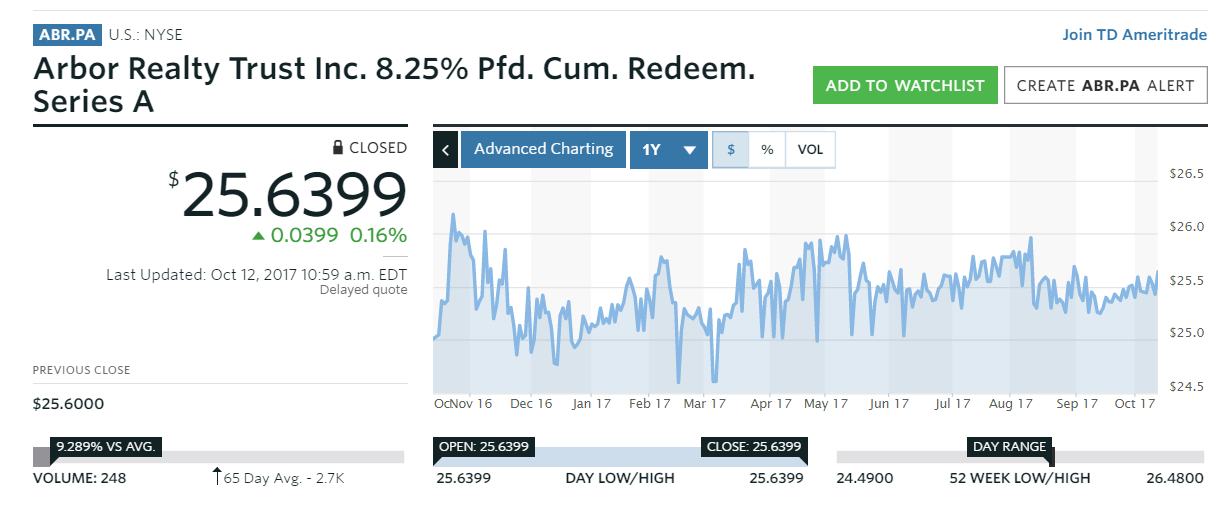The image is a horizontally rectangular screenshot from an investment platform listing specific details about a company. 

In the upper right corner, there's a call-to-action reading "Join TD Ameritrade." The top left corner displays the company name and security details: "Arbor Realty Trust, Inc. 8.25%, PFD, CUM, Redeem. Series A." Adjacent to that, there are two buttons labeled "Add to Watchlist" and "Create ABR.PA Alert."

On the left side of the screenshot is the price information for the listed security. The current price is noted as $25.6399, which marks an increase of $0.0399, or 1.6%. This information was last updated on October 12th, 2017, at 10:59 a.m. Below this, the "Previous Close" is indicated as $25.6000.

To the right of the price details, there's a graph charting the stock's performance over the year, with dates ranging horizontally from October 2016 to October 2017. The vertical axis on the right and bottom of the graph displays share prices, starting at $24.5 at the bottom and reaching $26.5 at the top.